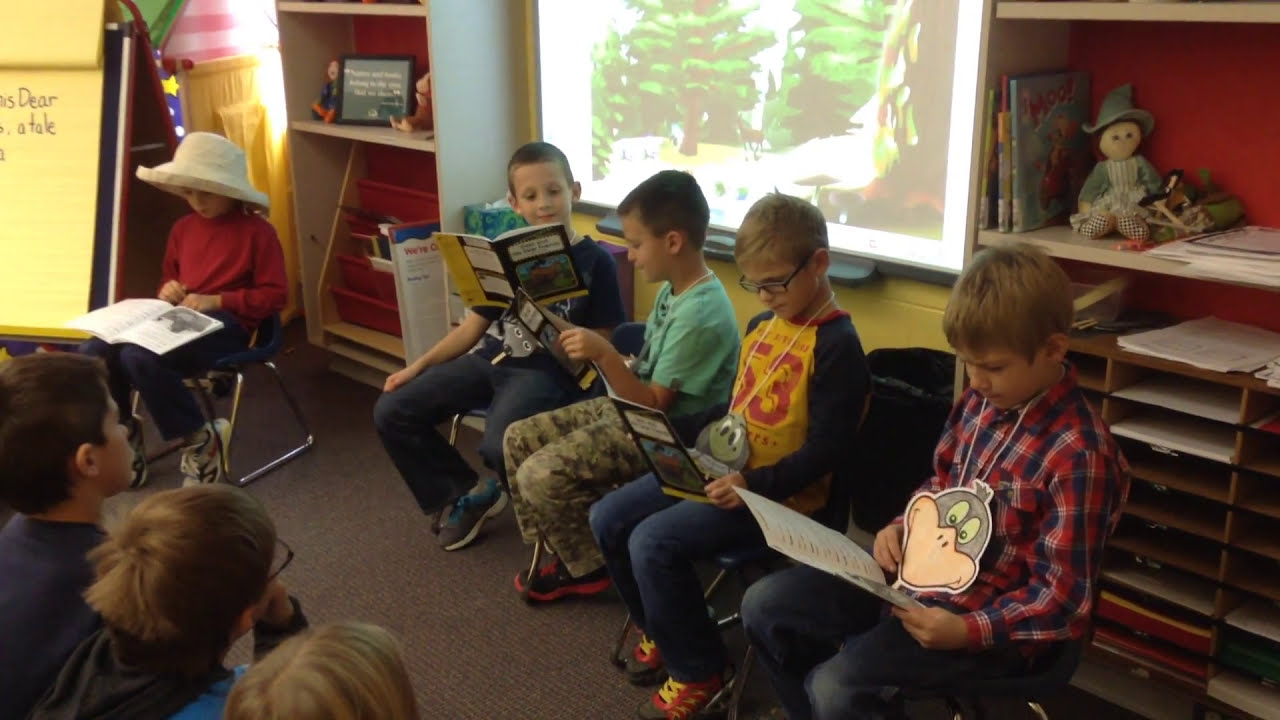In this detailed photograph taken inside a brightly lit elementary school classroom, likely a library, a small group of first or second graders is deeply engaged in reading. At the center of the image, four boys sit in a row. From right to left, the first boy wears a red plaid shirt, the second a bright orange shirt with the number 53 in red, the third dons a green shirt paired with camel pants, and the fourth, dressed in a black t-shirt and pants, holds an open book. Each boy sports a lanyard with a name tag. Facing them to the left are three more children, mostly visible from the tops of their heads. Among these three, the focus is drawn to a little girl in the far left, distinguished by her oversized straw hat, red shirt, and black pants, as she reads a book placed on her lap. Behind the group of boys, the classroom wall features a window shaded with an illustration of a deer in a forest, permitting streams of natural sunlight to illuminate the scene. Flanking this window are shelves filled with books and various educational materials. An easel with large sheets of paper is visible to the left, displaying the words "deer" and "tail." In the background, a TV screen projects a serene forest scene, reinforcing the educational and explorative atmosphere of the room.